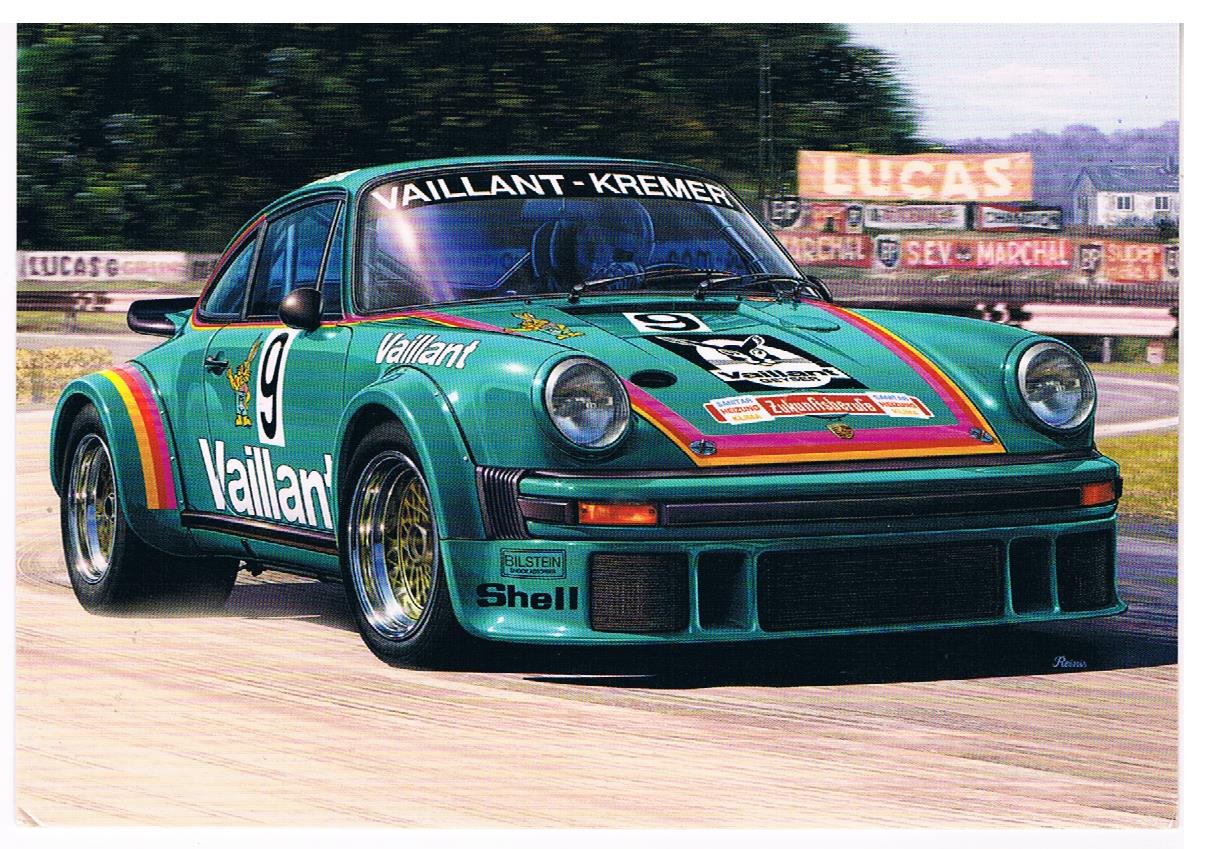This detailed, artistic drawing depicts a teal green Porsche race car navigating a racetrack. The car, adorned with numerous advertisements, features the prominent black number "9" on a white rectangle on its left passenger door, just above the bold white letters spelling "Valiant". The front hood displays a vertical column of ads, including a partially obscured company logo starting with a "V" and an ad for Valvoline. "Valiant-Kremer" is printed in white on a black strip across the top of the windshield.

The Porsche's front bumper is black with yellow horizontal turn signals, and its distinct bug-eyed headlamps are typical of the brand. The front spoiler, resembling a chainmail design with rectangular cutouts, bears the names "Bilstein" and "Shell" in black font on the far left. The rear wheels feature a unique multicolored striping pattern in red, yellow, and green, complemented by gold rims.

In the blurred background, a heavy treeline frames the racetrack, accompanied by a series of banners advertising "Lucas Oil," "SEV Marshall," and "Champion". The grayish-white track encircled by a steel guardrail completes the setting, along with a distant white house with windows and a gray roof visible in the upper-right corner. The dynamic composition and attention to detail suggest the car's motion towards the right, contributing to the overall sense of speed and competition.